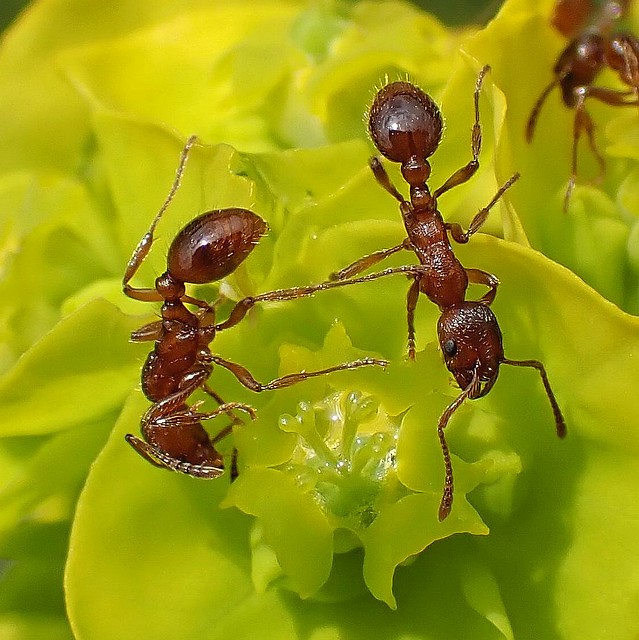In this hyper-realistic, up-close image, three reddish-brown ants are seen crawling on vivid yellow-green blossoms. The two prominent ants, positioned in the foreground, exhibit remarkable detail, including the fine hairs on their abdomens and their tiny pincers near the flower's center stamens. They are observed from different angles, with one viewed from the side and the other from above, both appearing to gather nectar. The third ant is partially visible in the blurred background, adding depth to the scene as it sits atop another flowering plant. Soft shadows cast by the central parts of the flowers indicate a blocked light source, enriching the image’s intricate textures and lifelike quality amidst the bright, lime sherbet-colored petals.